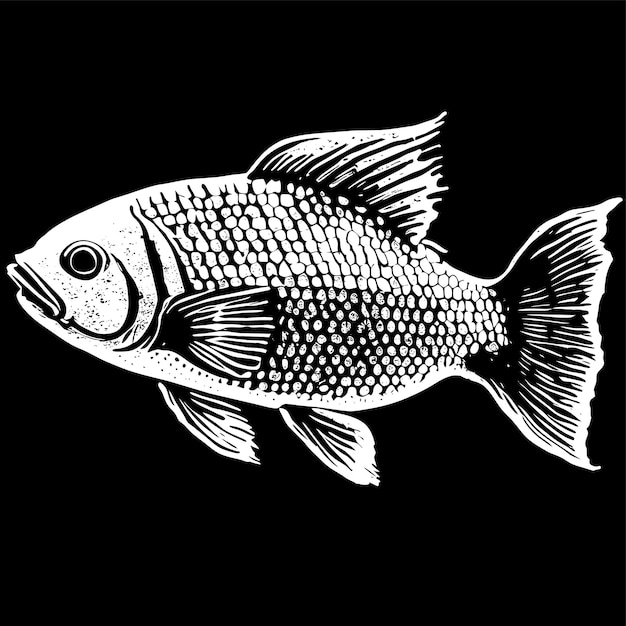This image features an artistic rendering of a fish, prominently displayed against a rich, very dark black background. The fish, possibly a goldfish or koi, is depicted in white with pronounced black scales and black outlining on the fins, creating a striking black and white contrast. The fish is oriented to face the left side of the image, which it spans horizontally from left to right and is centered vertically within the square format. It showcases a typical structure with one large dorsal fin on top, two lower fins, a central fin, and a tail fin, alongside a visibly large eye and mouth. The style of the rendering resembles a lithograph print, emphasizing the detailed scales and fins against the stark black backdrop, bringing out the intricate details and the neutral expression of the fish.